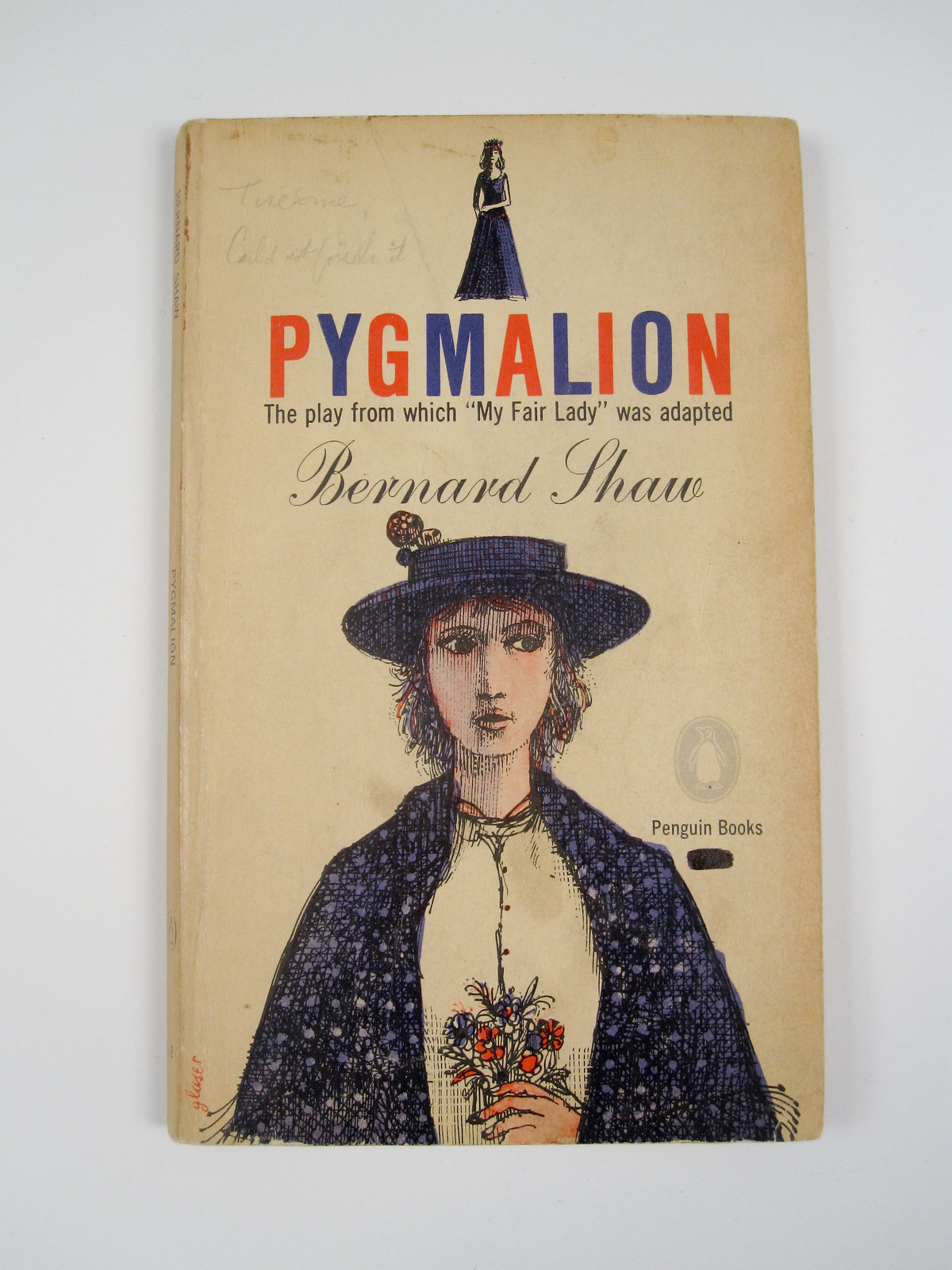The image is a color photograph of a vintage book cover set against a light blue background. The cover, with a slightly faded beige and tan color, showcases an illustration in black and white with accent colors in red and blue. Dominating the top half of the cover is an image of a woman in an old-fashioned, long blue dress and a hat with a blue rim. She is wearing a blue overcoat and a white blouse and holding a bouquet of flowers in front of her chest while looking to the left with a worried expression.

The title "Pygmalion" is prominently displayed in bold, alternating red and blue letters. Below the title, black lettering states: "the play from which 'My Fair Lady' was adapted." The author's name, Bernard Shaw, appears in black cursive script further down. Positioned on the cover above the title is a smaller picture of the same woman, emphasizing the vintage style of the book.

A Penguin Books logo is set on the bottom right corner, indicating the publisher. The overall design and imagery evoke a sense of nostalgia, indicative of a classic literary work.